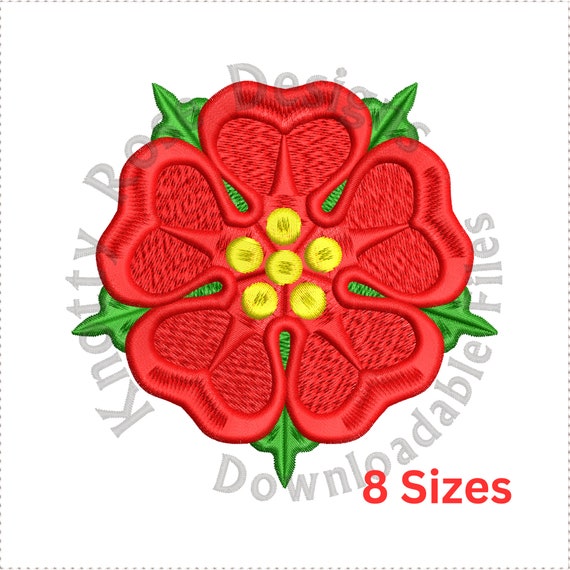This detailed photograph appears to be a promotional image for "Knotty Rosa Designs," specifically advertising downloadable files available in eight different sizes. The design showcased is a striking 3D-like embroidered red flower patch, ideal for application on garments like shirts. The flower features five heart-shaped petals, bright red in color, emanating from a central point. Between each of these petals, there are vivid green leaves, giving a balanced aesthetic to the arrangement. At the heart of the flower, six small yellow circles are evenly distributed, representing the stamen. The entire design exudes a three-dimensional woven texture, despite being a flat image. The text on the photograph emphasizes the downloadable nature of the files, making it clear that the design can be replicated in various sizes. The promotional frame around the image, marked by a dotted line, further accentuates the professional and polished presentation, suggesting it might be something available for purchase on platforms like Etsy.